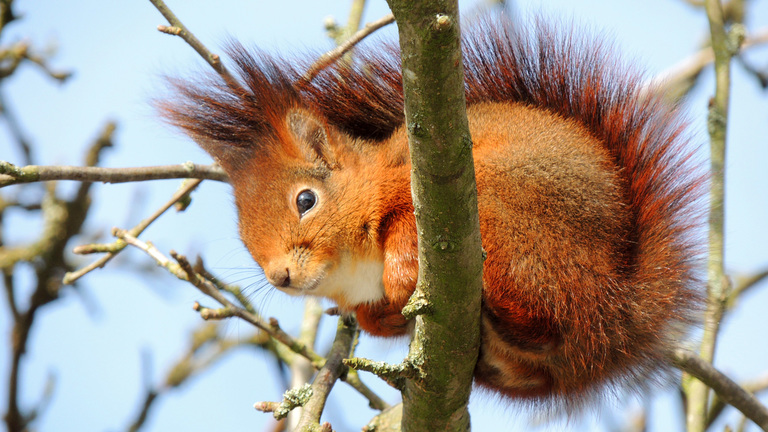Perched on a thick, leafless branch in a tree, a small, uniquely adorned squirrel commands attention with its striking appearance. This reddish-brown creature, with fur ranging from orange to dark brown, sports an impressive mohawk that runs from the top of its head straight down the middle of its back to the tip of its tail. The fur is spiked and vibrant, creating a striking contrast against the cyan, blurred sky in the background, which hints at a mid-morning setting. The squirrel is crouched low, legs tucked closely together under its small body, and its tail wraps snugly around its spine. Long hairs around its ears add to its distinctive look. The squirrel, unaware of the camera, looks downward with one visible dark eye, black nose, and tan underfur peeking out beneath its chin. The surrounding branches, devoid of leaves, suggest a winter season or the transition from spring, framing the focal point of this captivating photograph.